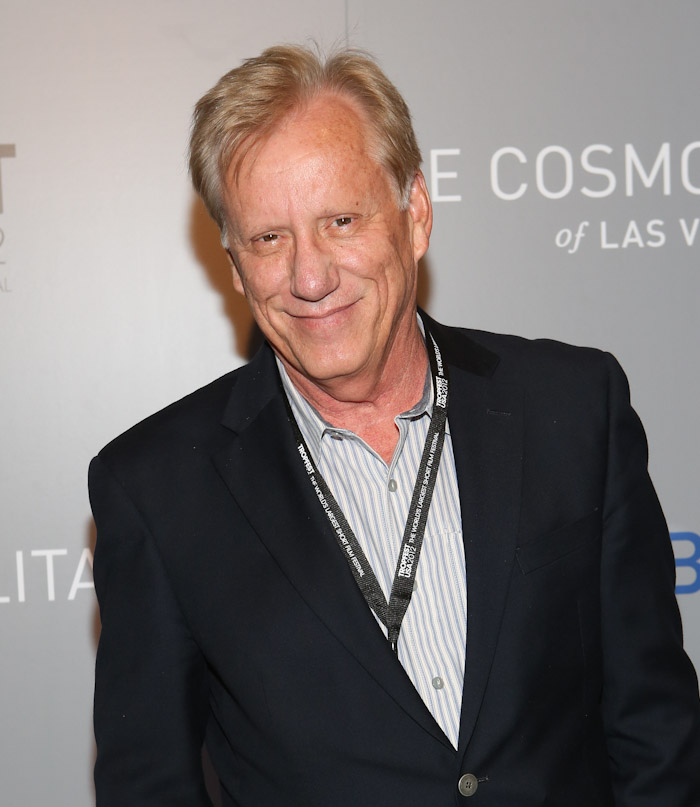The image features James Woods, a well-known actor, who appears to be in his 60s based on his grayish-brown medium-length hair. He is at an indoor event, wearing a black suit jacket buttoned near the navel over a light blue and white striped button-up shirt. Around his neck, there is a black lanyard with the year "2012" visible, suggesting the photo might be from that year or shortly thereafter. James is smiling directly at the camera, giving a sense of warm engagement. The background showcases a wall poster or wallpaper with somewhat obscured text that reads, "The Cosmo of Las Vegas," accompanied by various logos. The high-definition quality and professional lighting highlight the detailed setting, making every element from the colors—gray, white, tan, black, and light blue—to the textures clearly visible.